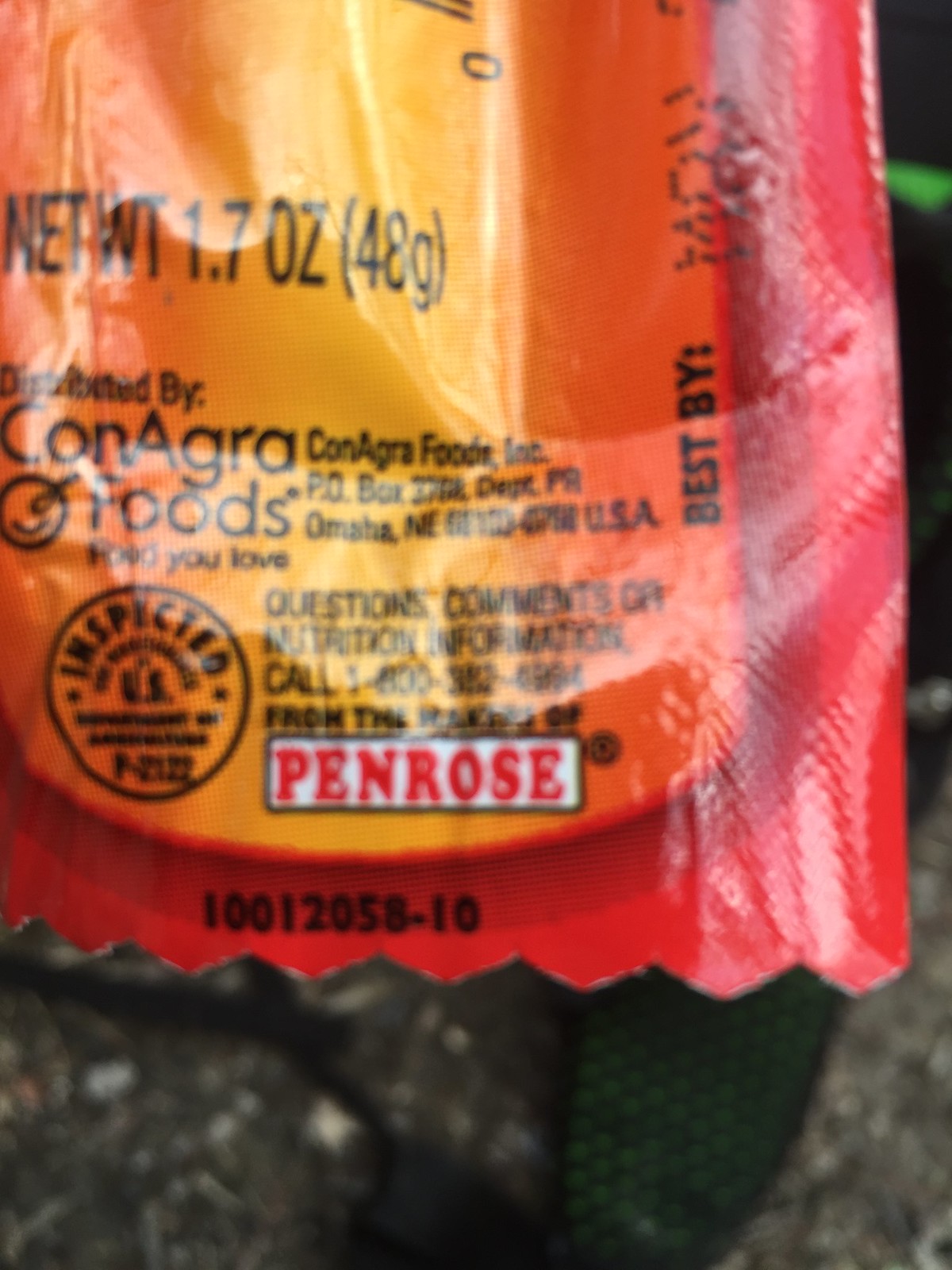The image is an up-close photograph of a food wrapper label, showing a brightly colored package with distinct red edges, an orange midsection, and a yellow-gold center. At the bottom of the packaging, "Penrose" is prominently displayed in red bold text within a white rectangle. Above "Penrose," there are instructions for questions, comments, or nutrition information, suggesting to call 1-800-382-0994. The top right corner indicates a "Best Buy" date that seems to be difficult to read, and the top left reads "Distributed by ConAgra Foods, food you love." The bottom left features an inspection mark. The wrapper's text also specifies a "net WT 1.7 ounces (48 grams)." The background shows a somewhat gray environment with a hint of green or black wheel-like structures, possibly amidst dark gravel, further indicating the snack or food packet is hanging in a setting that is not completely clear.